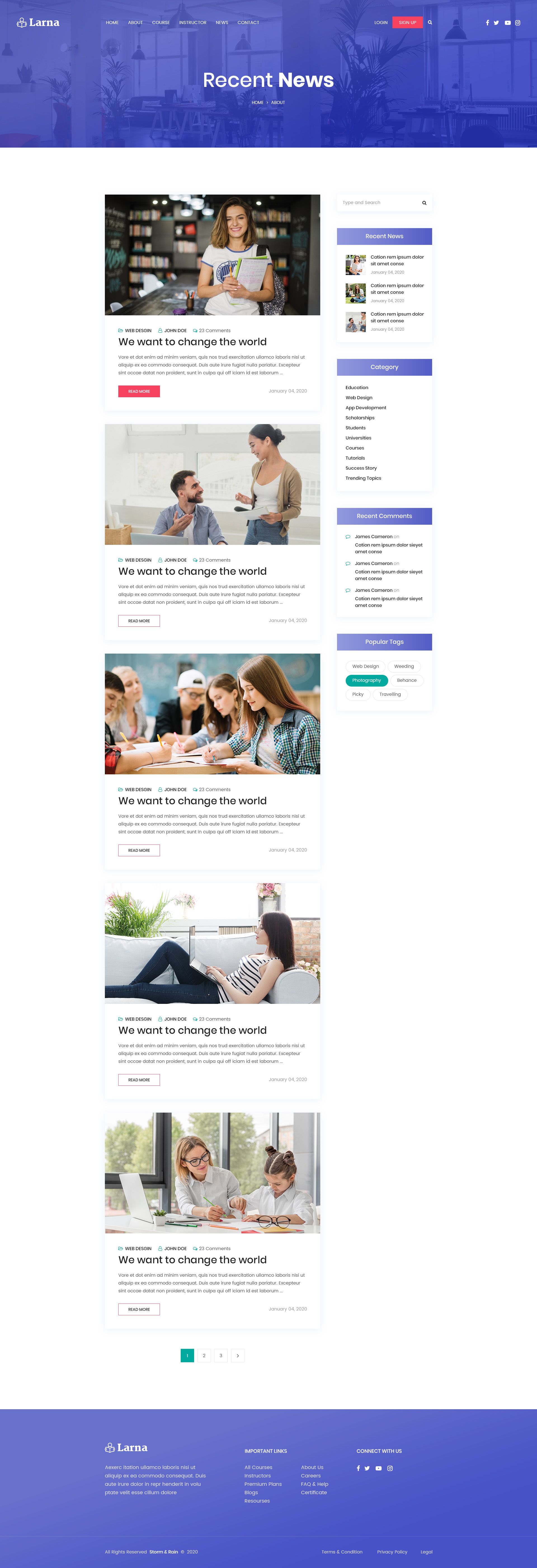The image appears to be a screenshot taken from a mobile phone, displaying a news app interface. At the top of the screen, there is a large blue rectangular banner with white text that reads "Recent News." Below this banner is a sizable white section containing five separate news articles.

1. **Top Article:**
   - **Image:** A female wearing a white shirt.
   - **Text:** A black headline followed by a short text description, although specific details are unreadable.

2. **Second Article:**
   - **Image:** A male sitting down while a female stands next to him, seemingly engaged in conversation.
   - **Headline:** "We want to challenge what works" is partially visible.

3. **Third Article:**
   - **Image:** Several young people, likely late teens or early twenties, sitting around a table.
   - **Headline:** "We want to challenge the world."

4. **Fourth Article:**
   - **Image:** A female laying on a couch.
   - **Headline:** "We want to change the world."

5. **Fifth Article:**
   - **Image:** A female sitting at a table with a little girl next to her.
   - **Headline:** Also reads "We want to change the world."

The recurring theme "We want to change the world" suggests a sense of activism or a call for transformative actions across different contexts in the displayed news articles.